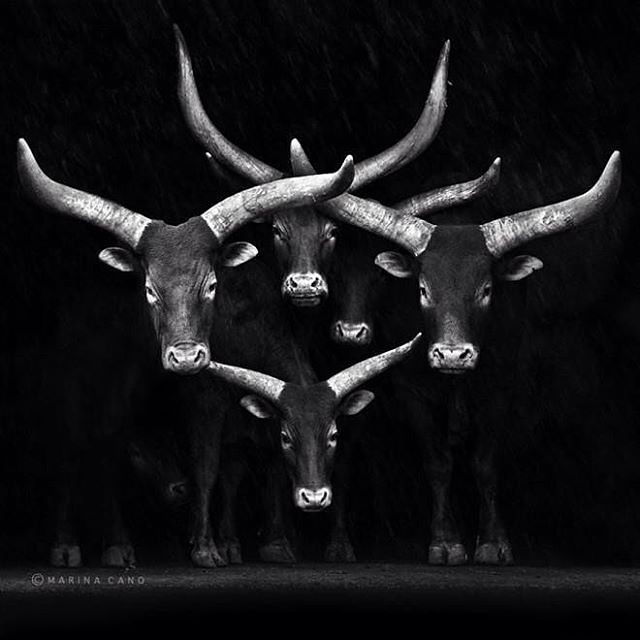In this evocative black and white photograph by Marina Kano, five oxen stand in a strikingly symmetrical formation, facing the camera directly. The image prominently features the heads and horns of four adult oxen, whose curved horns extend sideways before pointing forward. A calf stands between these adults, positioned in the middle, bottom section of the frame. Another adult calf is visible behind and to the left of the central ox. The dark background, coupled with the snowfall drifting from the top left corner, adds an eerie, almost surreal quality to the scene. Text at the bottom left corner reads "Marina Kano," asserting the artist’s copyright on the image.